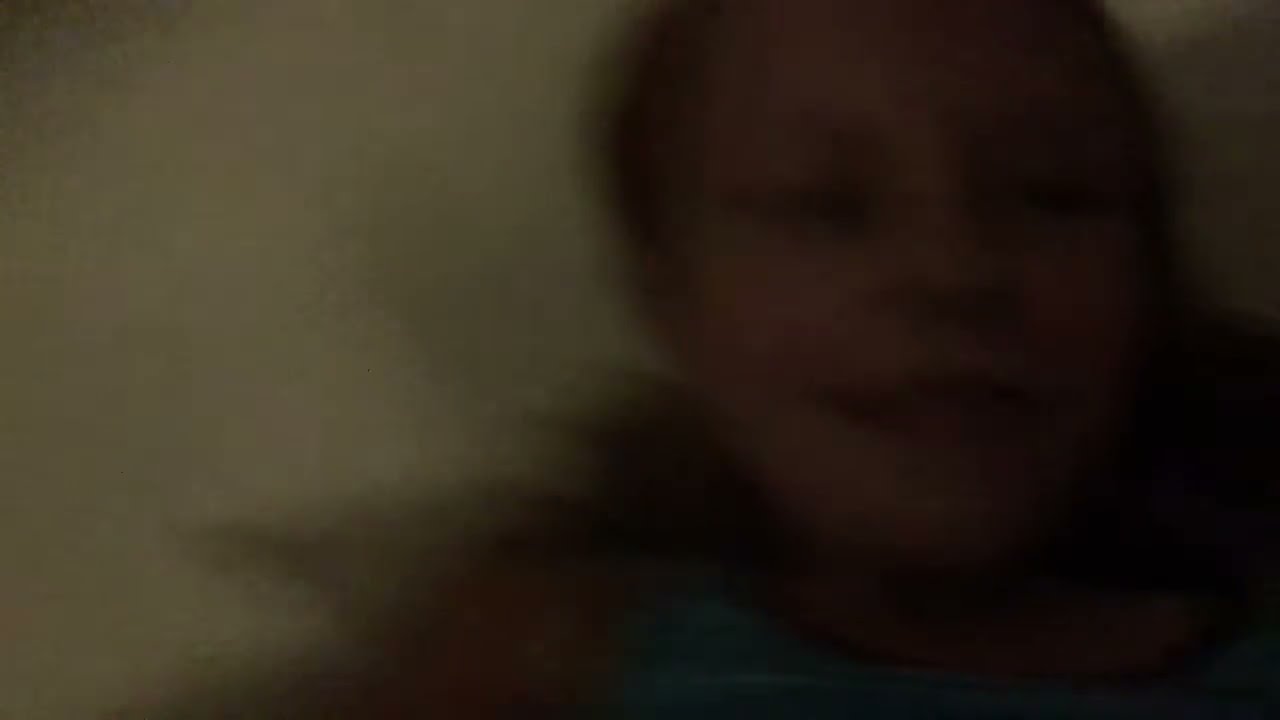The image is an extremely out-of-focus, low-light photograph that captures a close-up of a young girl's face occupying slightly more than the right half of the frame. She appears to have long, dark hair reaching her shoulders and is wearing a blue sleeveless shirt. The girl's face is just starting to form a smile, but her facial features, including her eyes, nose, and lips, are very blurry and indistinct. The left half of the image is dominated by a dark gray or brownish-white background, possibly a wall. The overall scene is so blurred and dark that it's difficult to determine whether the girl is standing, sitting, or laying down.